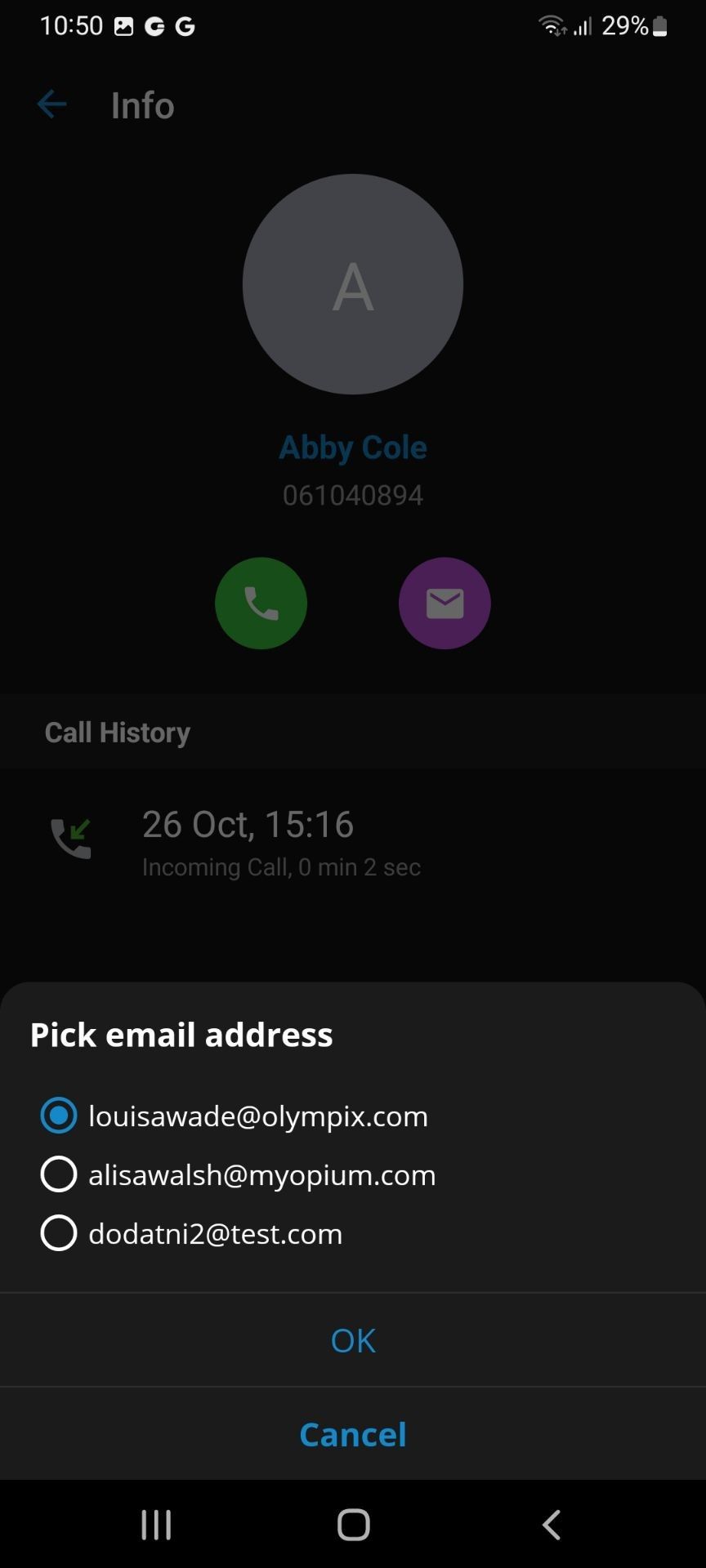The image displays the interface of an Android device. Key UI elements indicating this include the three vertical lines on the bottom left, followed by a square symbol, and an arrow pointing left. The device time at the top is 10:50, and there are notifications including an image and two from Google. Signal indicators show two out of four Wi-Fi bars and three out of four cellular bars, with the battery level at 29%.

The screen centers on a contact update for Abby Cole, denoted by a gray circle with a white "A" and the number 0610894. Options for contacting Abby via a green circle (phone) and a purple circle (email) are visible. The contact history shows an incoming call from Abby on October 26 at 15:16, lasting 2 seconds, possibly indicating an accidental call.

The primary action involves selecting an email address for Abby from a list, which includes "Louisa Wade at olympix.com" (misspelled as olympics), "Alyssa Walsh at myopium.com," and "doe.ni2 at test.com". At the bottom, options to confirm or cancel the selection are provided, suggesting the user is updating Abby Cole's email address.